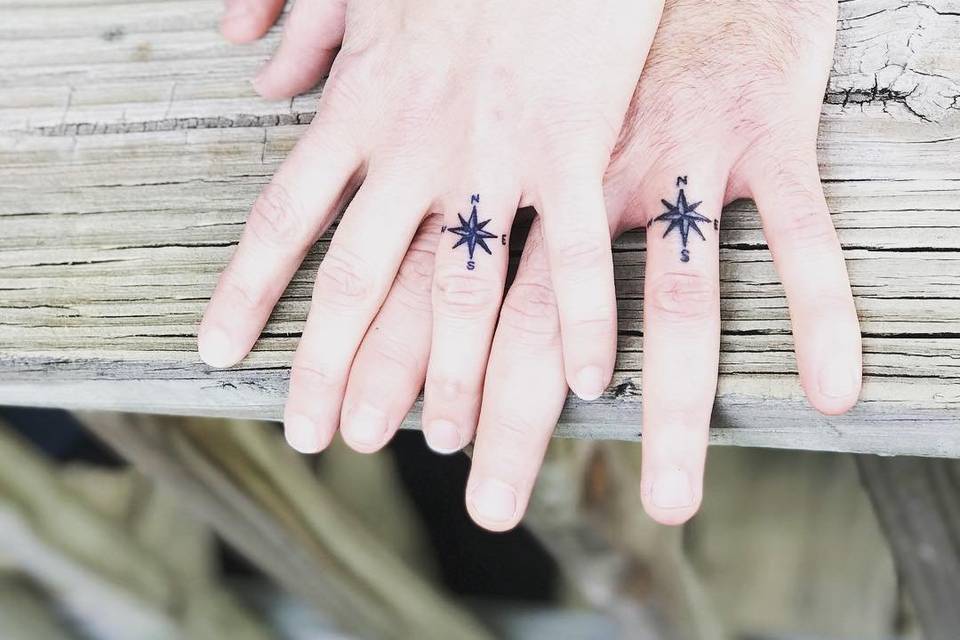In this image, we see a couple's left hands resting on a worn wooden board, possibly part of a hiking trail bridge. Their hands are not fully holding but are instead layered, with his hand underneath and her hand on top, fingers gently intertwined. Both individuals proudly display matching compass tattoos on their ring fingers, each compass featuring the cardinal directions (N, E, S, W) as well as the intercardinal points. His hand, slightly more hirsute and with noticeably longer fingers, provides a size contrast to her more delicate hand. The close-up shot captures the intimate detail of their connection and shared ink, symbolizing their mutual direction and journey together.